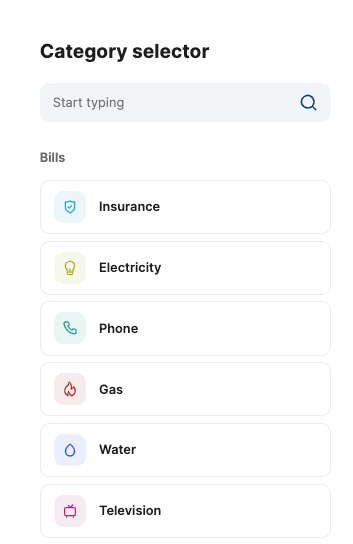This image is a vertical smartphone screenshot with a white background. At the top, bold black text reads "Category Selected, Selector." Just below this header is a light gray rectangle with rounded corners, containing the placeholder text "Start typing" in gray font, accompanied by a gray search icon on the right side—a circle with a small diagonal line extending downwards to the lower right.

On the left side within this gray rectangle, "Bills" is written in black font. Below this input area, there are various categories enclosed in thinly outlined rectangles. From top to bottom, the categories are listed with their corresponding icons: 

- "Insurance" (icon not described)
- "Electricity," accompanied by a light bulb icon
- "Phone," paired with an image of a phone receiver
- "Gas," illustrated with a flame icon
- "Water," indicated by a droplet of water 
- "Television," represented by a square with rabbit ears on top, symbolizing a TV